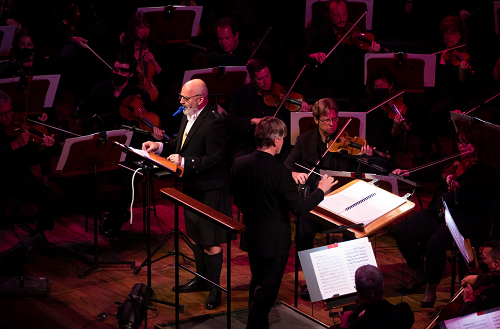In the image, a musical orchestra is performing, featuring two conductors. Both conductors are dressed in black suits. The conductor on the left is bald, wears glasses, and has a white beard. He stands facing outwards towards the audience, with a blue object in his mouth, and is positioned in front of a podium with a piece of paper. The conductor on the right has short hair with some gray, or salt-and-pepper tones, and also faces his respective side of the ensemble. The lighting highlights these two conductors, making them the focal point of the image.

Behind and around the conductors, numerous orchestra members are seen playing various instruments, predominantly violins. To the top left, one musician is playing what appears to be a cello, while other violinists are clearly visible on the right-hand side and in the first two rows. The scene suggests a larger orchestra, with an estimated 10 to 15 visible members, including both men and women. Music sheets, some highlighted, are discernible in front of select musicians, adding to the intricate details of the performance setup.